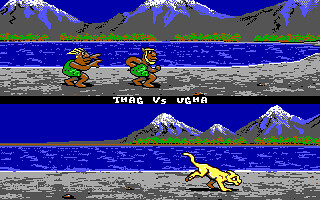In this scene from an older video game, two cavemen characters, Thag and Ugma, are depicted running on a gray dirt path. Set against a detailed backdrop, the imagery includes green grass, a royal blue sky, mountains capped with snow, and a body of water. The two cavemen are shown in green shrouds, resembling little islanders with straw hats and bare legs. They appear to be in a chase, pursued by a small yellow dinosaur-like creature. The path they are running on is paralleled by a log over the water, adding to the adventure theme. The title "Thag versus Ugma" is prominently displayed in the middle of the screen, suggesting a competitive or confrontational element to the scene.